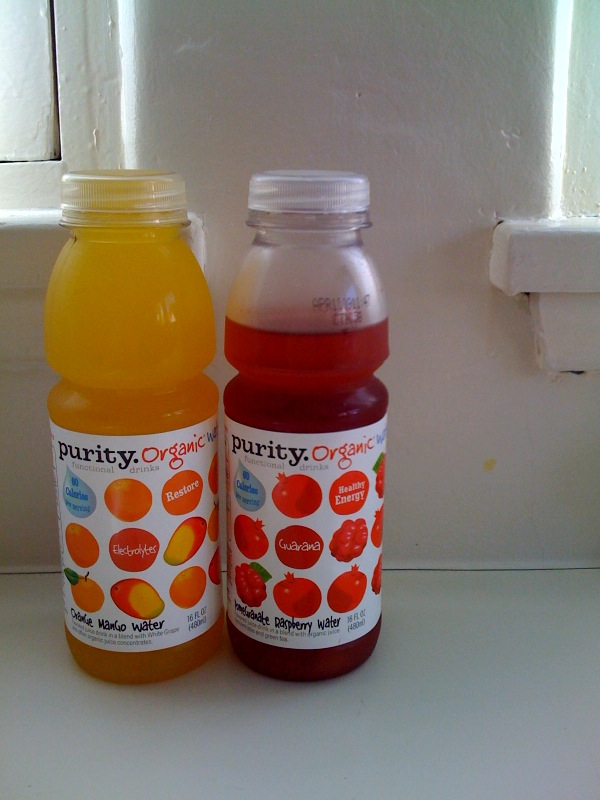In this photograph, two bottles of fruit-infused beverages are prominently displayed against a plain white background. The setting includes a white surface and a wall, presumably painted several times over as indicated by its notably thick texture, although this backdrop does not detract from the focal point: the drinks.

The beverage on the left is a striking shade of orange, suggesting a flavor profile of citrus and tropical fruits. The label reads "Purity Organic Restore Electrolytes Orange Mango Water." This label, adorned with playful, cartoon-style fruit illustrations, stands out against its white background. The bottle appears unopened, filled to the brim with its vibrant liquid.

To the right is a second bottle, this one a deep berry hue, indicative of a berry-based flavor. The label identifies it as "Purity Organic Healthy Energy with Guarana," although some specifics remain partially obscured. It likely mentions “Raspberry Lemonade Water.” This bottle has been opened, evidenced by a slightly elevated cap and the liquid level sitting about an eighth of the way down. Both bottles contain 16 ounces of refreshing, fruit-flavored hydration.